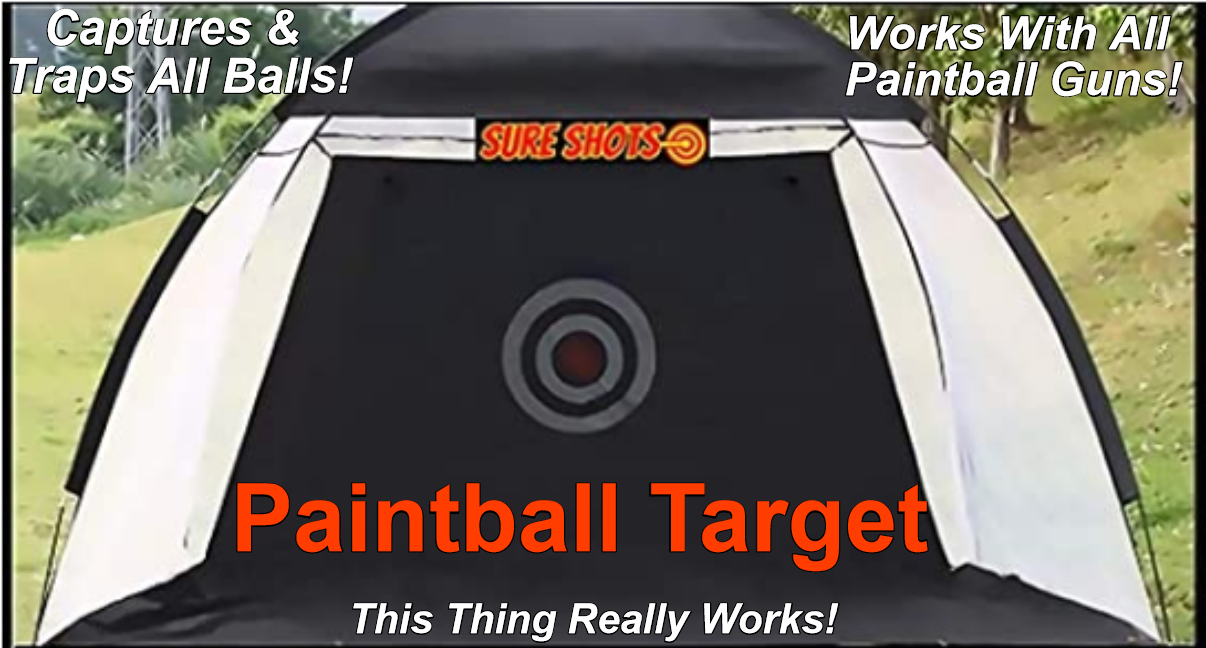The image is an advertisement for a paintball target called "Sure Shots," prominently displayed in the center. The target is integrated into a black and white tent-like structure with an open front designed to capture paintballs. The center of the target features a gray bullseye with a dark red center. Text on the top of the tent reads "Sure Shots," and beneath it, "Paintball Target" is written in red. The phrases "This thing really works" and "Captures and traps all balls" are visible on the top left, while "Works with all paintball guns" is seen on the top right. The setup is located in a park-like area, with lush green grass in the foreground and trees and bushes in the background. A radio tower or telephone pole is faintly visible on the far left side.